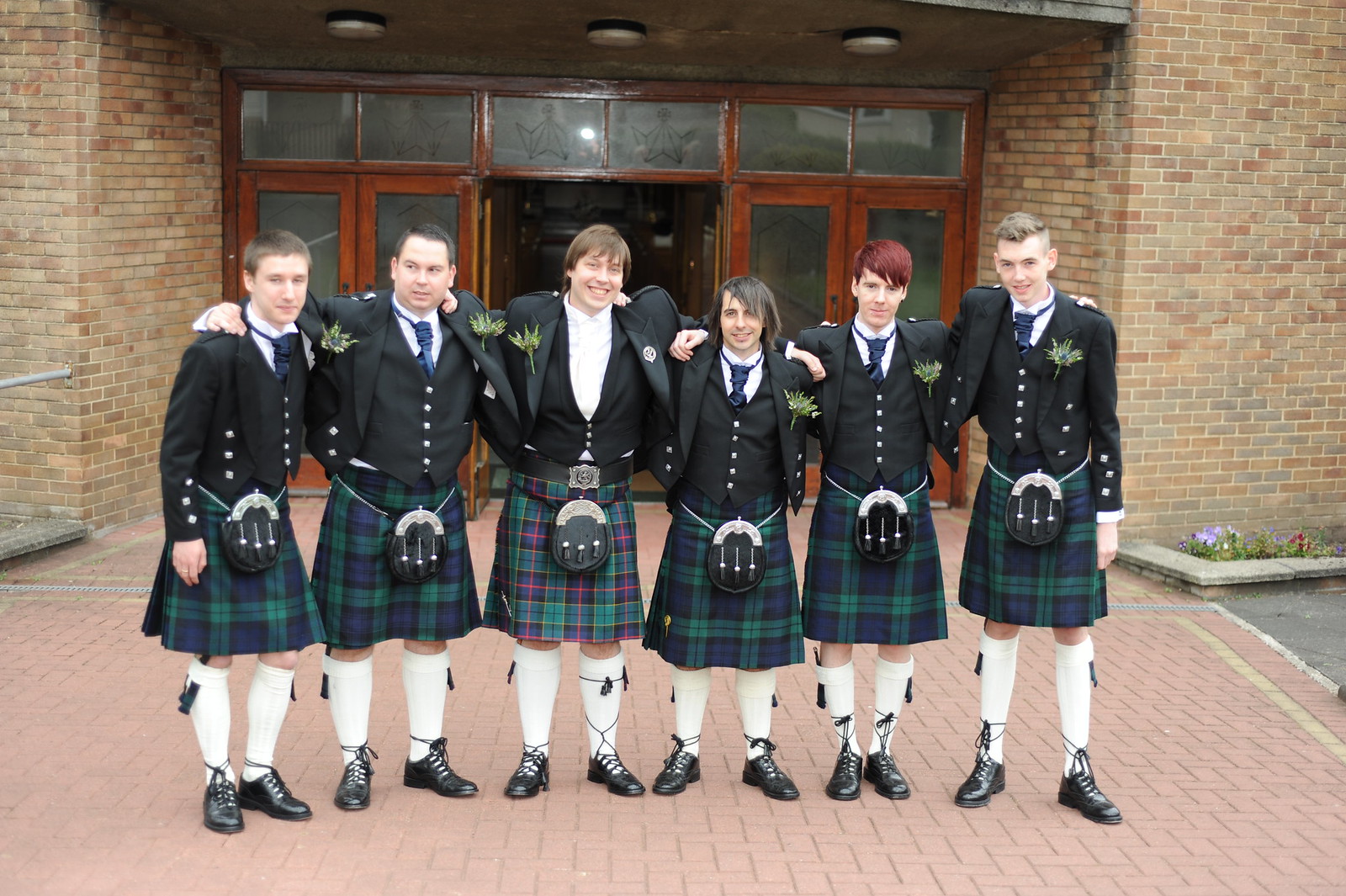In this detailed image, six young males are standing in front of a distinguished brick building, possibly a school or church, with wooden-framed doors that are open behind them. Each of the boys, who range in age from their mid-teens to their mid-to-late 20s, is dressed in traditional Scottish attire. They are wearing green and navy blue kilts paired with black jackets, vests, and white button-up shirts. High white knee socks and polished black dress shoes complete their outfits. A small traditional sporran, a type of pouch, hangs from the front of each kilt. Each boy also sports a boutonniere on his jacket. They stand together on a red brick walkway with their arms linked, all smiling warmly at the camera, conveying a sense of unity and camaraderie. The group includes boys with different hair colors—one with bright red hair and another with blonde, while the rest have brown hair. The full length of their bodies is visible within the center of the image.